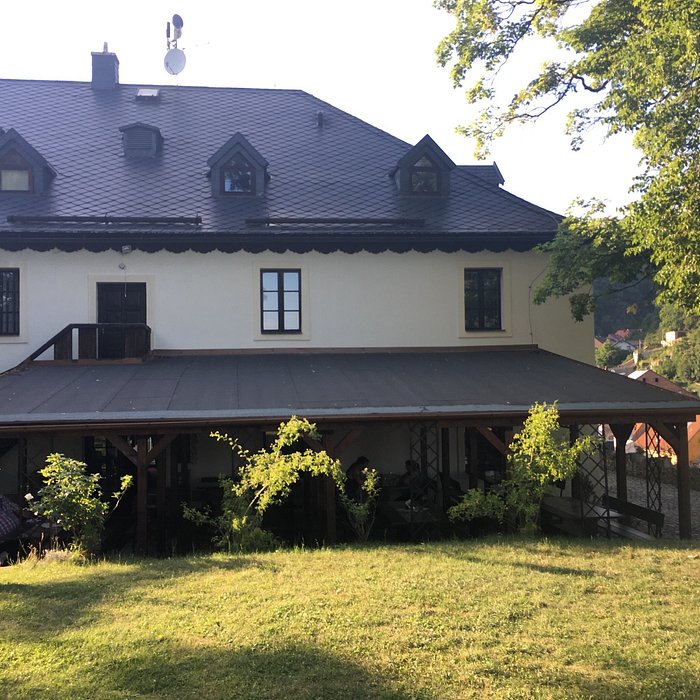The photograph showcases a white stucco house with a dark, almost black, possibly charcoal-colored or blue tile roof. The two-story structure features an upper level with dark brown wooden-framed windows and a very dark brown wooden door. A set of stairs leads down from a door to an open but shaded porch area, supported by wooden columns. Under this canopy, several wooden tables and benches are arranged, where people are dining comfortably, suggesting that the establishment might be a restaurant. The foreground displays lush green grass, illuminated by sunlight, with a few shrubs. The scene hints at a spring or summer setting. There are green trees with leaves and a stone walkway visible to the right. Additionally, parts of a village with other houses and roofs can be seen in the background under a cloudy, overcast sky.